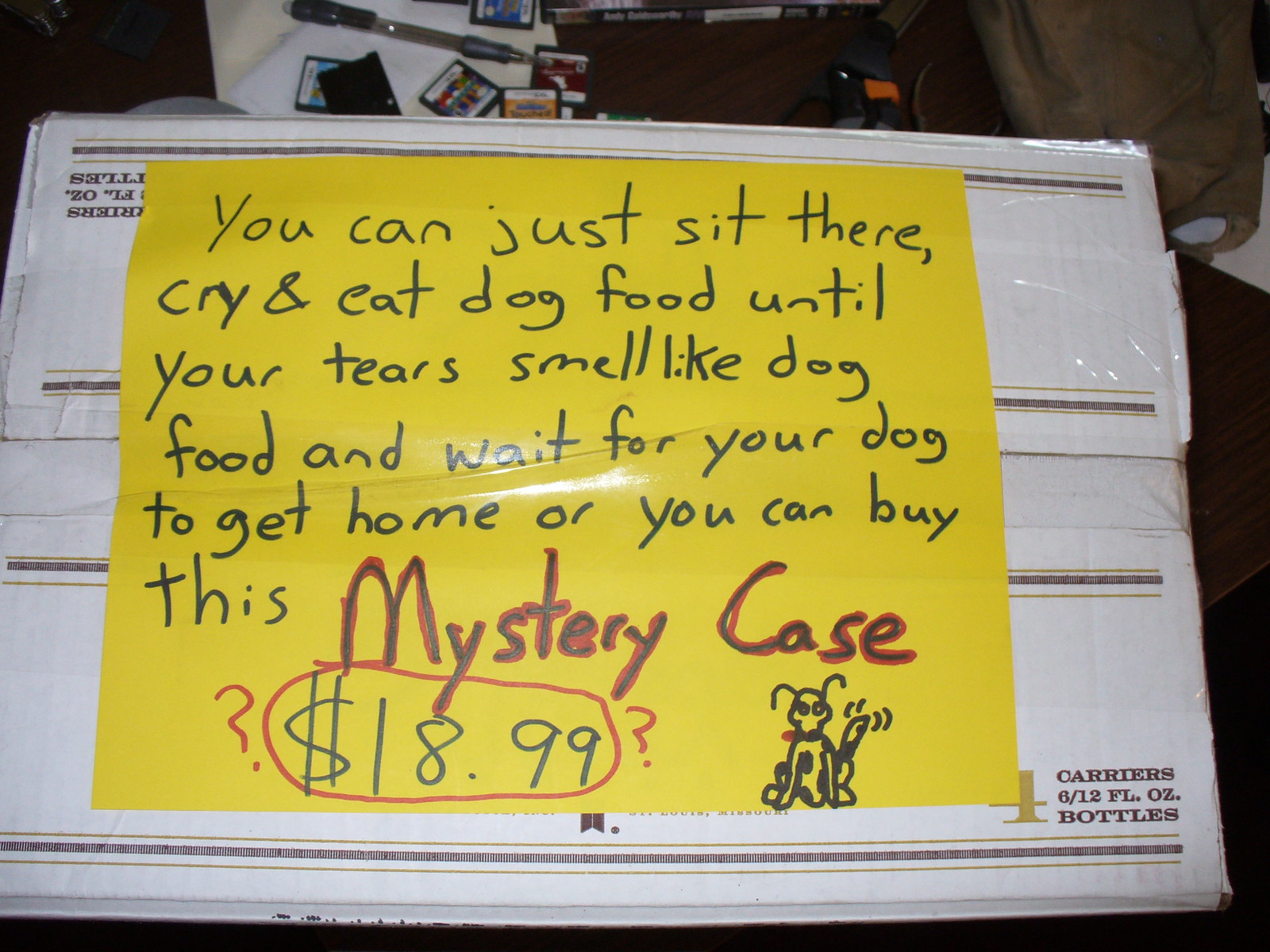The image is a full-color photograph taken indoors, depicting a handmade sign prominently displayed atop a white cardboard box sealed with tape. The box is partially wrapped in plastic and features printed text in the lower left and upper left corners that reads "4 carriers, 6/12 FL OZ bottles." The main focus of the photograph is a bright yellow piece of paper positioned on top of the box. This yellow paper, slightly covered in plastic, exhibits visible wrinkles reflecting light.

Handwritten in black marker, the sign humorously reads: "You can just sit there and cry and eat dog food until your tears smell like dog food and wait for your dog to get home, or you can buy this." This message is followed by "mystery case," highlighted with red marker. Below "mystery case," a small drawing of a black-and-white spotted Dalmatian wearing a red collar adds a playful touch. Accompanying the text, a price of "$18.99" is boldly written, bracketed by red question marks, and circled in red for emphasis. In the background of the photograph, a pen or pencil and several small disc-like objects are also visible. The creative and cheerful tone of the sign suggests it was crafted to evoke curiosity and amusement.